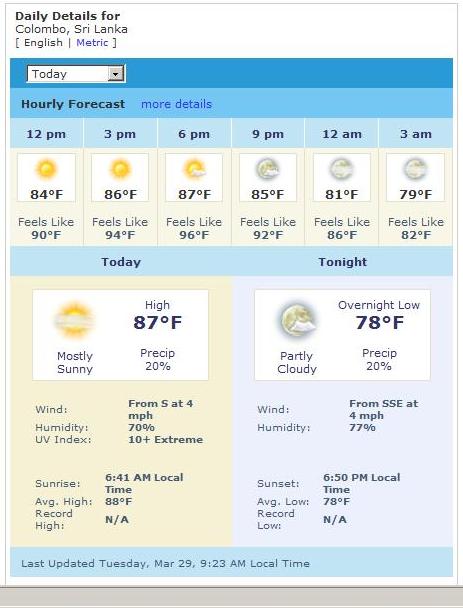The image displays a weather application screen, likely on a tablet or a wide smartphone. 

**Header:**
- The top section of the screen features a white background with bold black text reading "Daily Details for", followed by lighter text indicating "Colombo, Sri Lanka". 
- Language and measurement systems are indicated, showing information in English and the metric system.

**Multicolor Banner:**
- Directly below, a multicolored banner indicates the weather section. 
- The upper part of the banner is a darker blue, possibly a navigation bar for selecting different time frames or specific days.

**Hourly Forecast:**
- Below the darker blue section is a lighter blue banner with bold text "Hourly Forecast". 
- A clickable "More Details" in blue suggests expanded information is available.
- The hourly forecast section displays weather predictions every three hours, rather than hourly, starting from 12 PM (noon) and continuing through 3 PM, 6 PM, 9 PM, 12 AM (midnight), and 3 AM.
- Temperature readings are as follows: 84°F, 86°F, 87°F, 85°F, 81°F, and 79°F, accompanied by corresponding "feels like" temperatures.

**Daily Forecast:**
- Further below, a detailed forecast for "Today" and "Tonight" is provided. 
- High and low temperatures, along with a consistent 20% chance of precipitation, wind conditions, and the times for sunrise and sunset, are included in this section.

The comprehensive layout offers a clear and detailed presentation of weather conditions in Colombo, Sri Lanka.